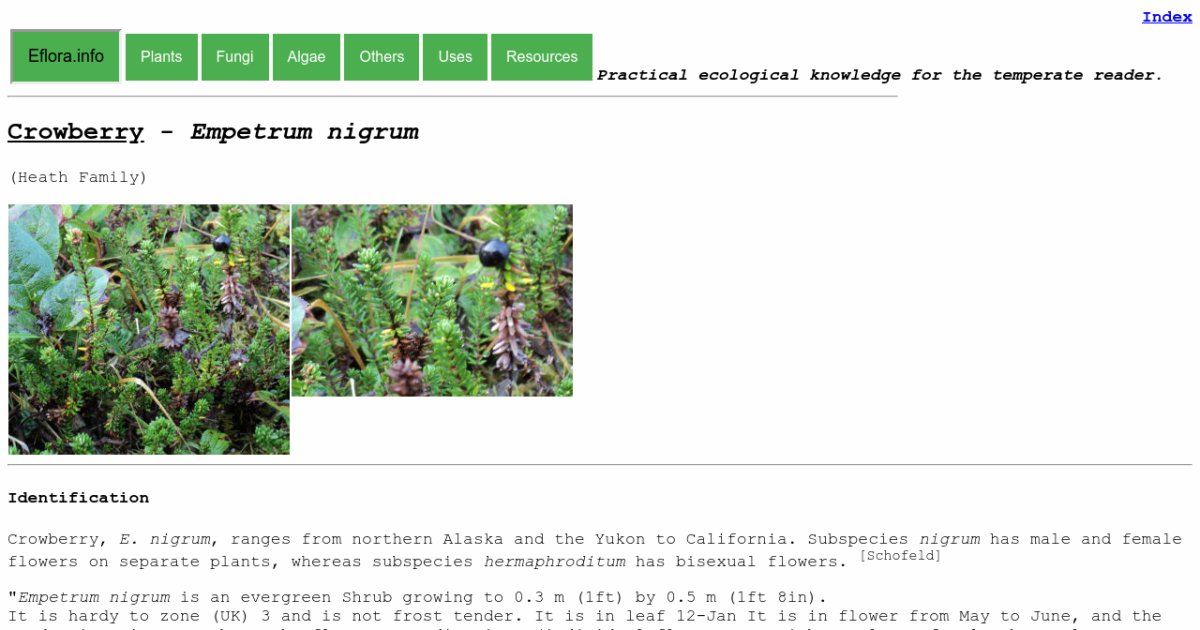The image depicts a detailed webpage primarily centered on a plant species, Crowberry (Empetrum nigrum), and features two side-by-side photographs of the plant. The top section of the page includes several green rectangular tabs with white text, arranged horizontally: "eflora.info," "Plants," "Fungi," "Algae," "Others," "Uses," and "Resources." To the right of these tabs is a horizontal line of black text on a white background reading, "Practical Ecological Knowledge for the Temperate Reader." Beneath this headline, a section starts with the title "Crowberry - Empetrum nigrum (Heath Family)," all in black text with Crowberry underlined. Following this, two images display close-ups of the Crowberry plant: the left image is a square frame showcasing green leafy vegetation, while the right image is a horizontal rectangle that includes some purple flowering elements among the green leaves, each topped with nearly black berries. Below the images is a section titled "Identification," though the specific text details here are unreadable.